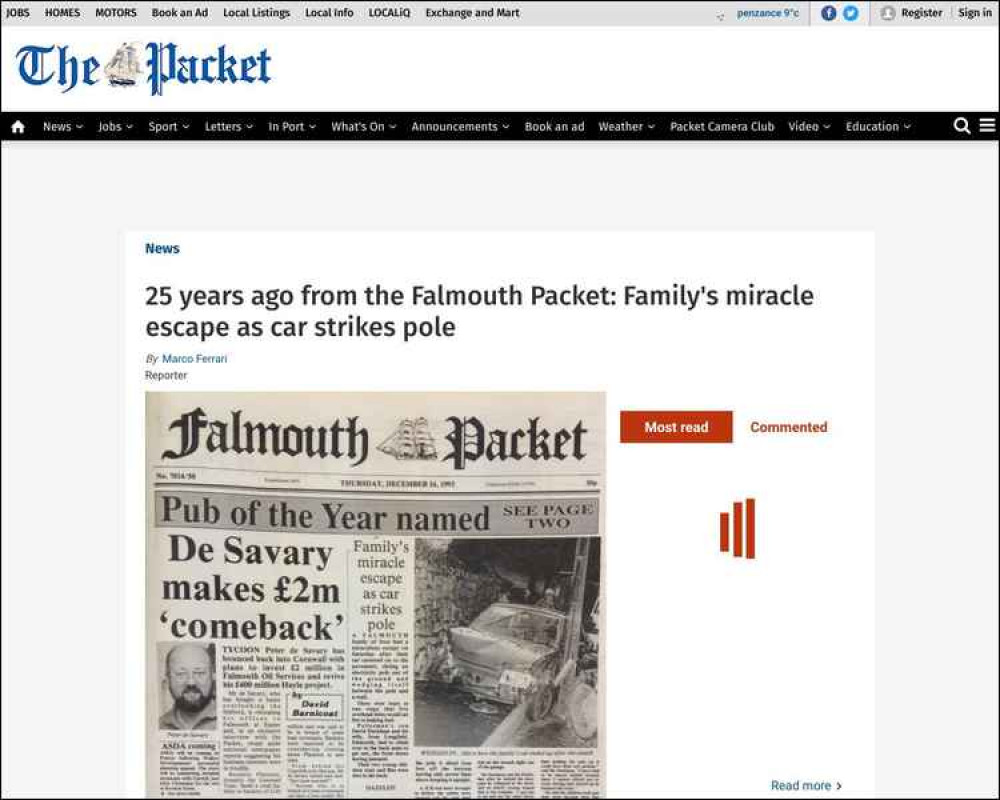This is a screenshot of a web page displaying a section of a newspaper. At the top of the page, there is a grey navigation bar with options for Jobs, Homes, Motors, Book an Ad, Local Listings, Local Info, Local IQ, Exchange, and more. On the right side of the bar, there is weather information indicating a temperature of 9 degrees Celsius, followed by icons for Facebook, Twitter, a person icon for account actions, and options to register or sign in.

Below the navigation bar on the left side, there is a blue script logo that says "The Packet" accompanied by an image of an old-time sailboat. Directly beneath this is a thin blue bar with various navigation icons and options including Home, News, Jobs, Port, Letter, Import, What's On, Announcements, Book an Ad, Weather, Packet Camera Club, Video, Education, and a search icon represented by a magnifying glass with three lines.

Centered below these navigation bars, there is the word "News" in small blue text. Underneath it, there is a headline in larger, bold black text that reads, "25 years old, Go from the Falmouth Packet, Family's Miracle Escape as Car Strikes Pole." The article is attributed to Marco Fiore, Reporter.

On the right side, there is a red box labeled "Most Read" next to a section titled "Commented." Below these sections, there are three thick red lines. In the bottom right corner of the image, there is a "Read More" button with a right-facing arrow.

The layout of the page is designed to provide quick access to various sections of the newspaper, with a clear focus on the featured article about the family's miraculous escape.